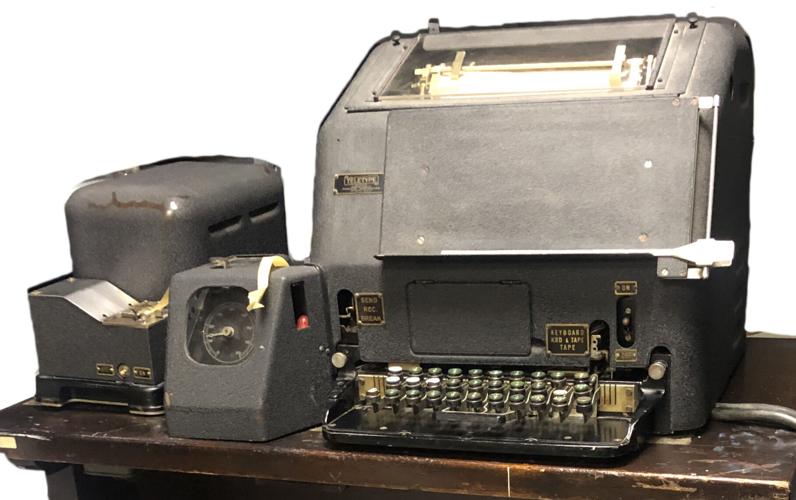This photograph, taken indoors and digitally altered to show only the essential details, features an old, worn, dark brown wooden desk with numerous chips and scrapes. Dominating the desk is a large, vintage, dark gray metal typewriter. The typewriter, located prominently on the right-hand side, boasts raised black, circular keys. At the top, the paper feeding mechanism is visible, with a lid that is currently open and hanging down.

To the left of the typewriter, two smaller gray machines occupy the desk. One of these machines has a visible gauge or dial on its front, suggesting it might be related to a timing or measuring function. The other device's purpose is less clear. The background of the image has been whited out, eliminating any distraction and putting all focus on this intriguing array of antiquated typing and possibly computational equipment.